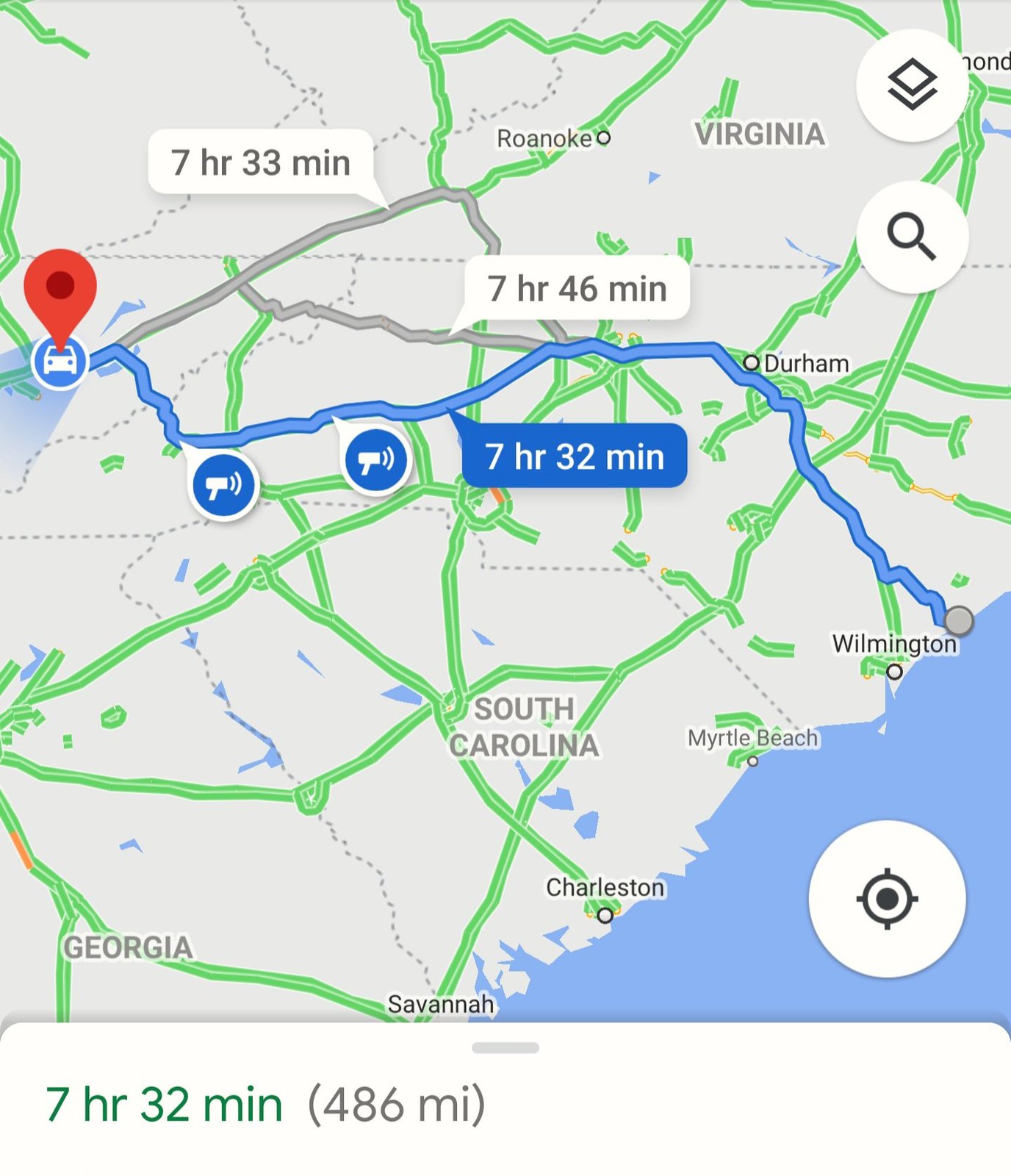This image is a detailed computer-generated map, resembling a Google Maps interface, showcasing a travel route on the East Coast of the United States. Highlighted in blue is the fastest route, taking approximately 7 hours and 32 minutes to reach Wilmington, which is marked as the destination. The journey originates from a location represented by a car icon, indicating the starting point. Two alternative routes are also displayed, one taking 7 hours and 33 minutes and the other 7 hours and 46 minutes. The total distance for the highlighted route is 486 miles. The map also includes surrounding states and nearby cities, providing a comprehensive view of the geographical context.